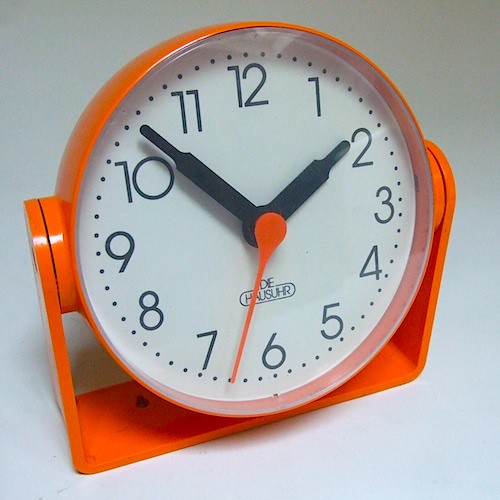A round clock with a white face is encased in an orange frame, prominently featuring the brand name "Dehauser" at the top left in black text. Black numerals from 1 to 12 are evenly spaced around the clock, marked by dots. The clock has three colored hands: the hour hand, pointing at 2, and the minute hand situated between 10 and 11, are both black. The second hand, which is orange, is positioned between 7 and 6. The clock's frame extends into two orange arms on the left and right, and a flat orange base at the bottom provides additional structure. A plastic cover over the clock face reflects some ambient light, while the floor underneath is white with noticeable scratches and a patch of gray in the top right corner.